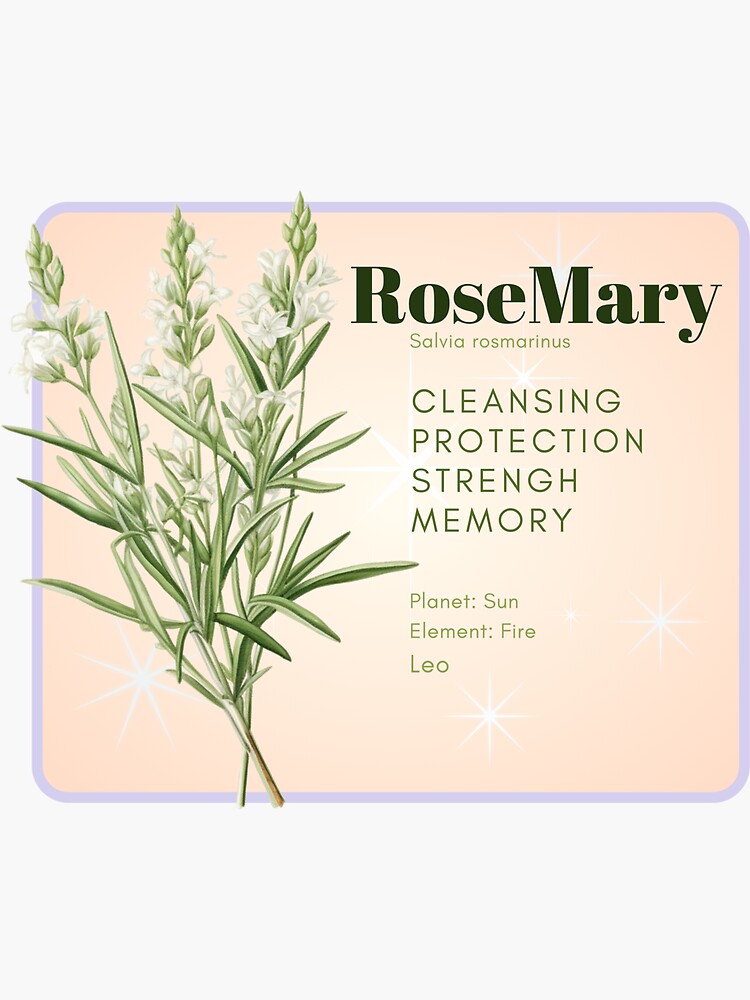The image showcases a detailed label, potentially for an organic health product, with a rosemary theme. Centered on the left side, it features a realistic illustration of a rosemary plant with two intersecting green stems, narrow, elongated leaves, and small white flowers each with five petals. Beside the plant, on the right side, the label includes descriptive text against a light peach background adorned with small star splashes. At the top, in large green letters, it states "Rosemary," followed underneath by its botanical name "Salvia Rosmarinus" in smaller green letters. Further down, a list of attributes is highlighted: "Cleansing, Protection, Strength, and Memory," also in green lettering. The bottom section of the label specifies astrological associations in smaller green letters, including "Planet: Sun, Element: Fire, Leo." Additionally, two large white stars and a smaller white star appear at the bottom right corner. The entire label is framed by a square with rounded corners and a light purple border, suggesting an elegant and holistic appeal typical for health-related products.